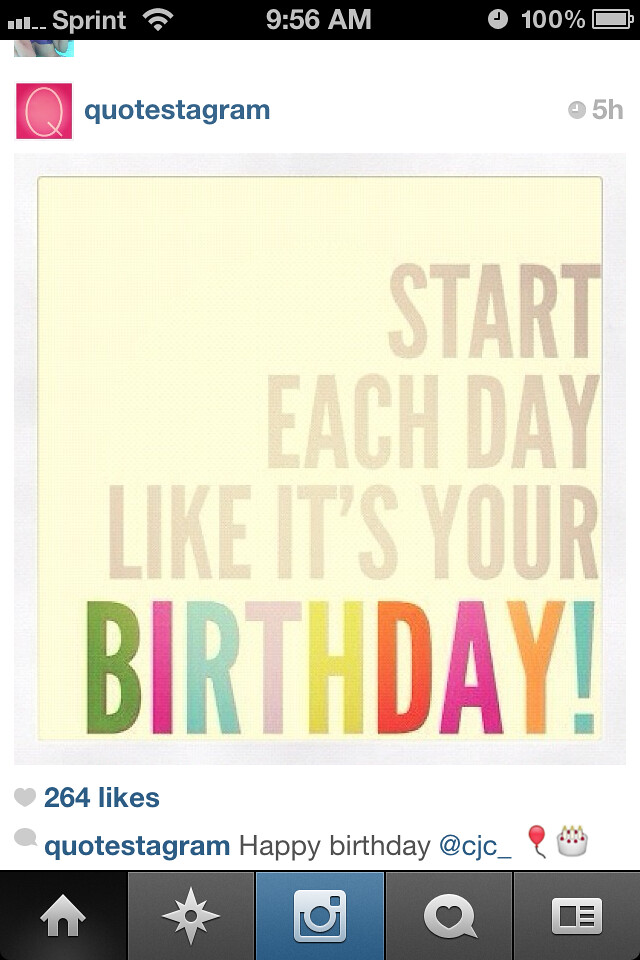This image appears to be a screenshot from a mobile phone displaying an app called Quote-stagram, possibly a spin-off of Instagram. The phone's status bar shows it's 9:56 AM, the carrier is Sprint, and the battery is at 100%. The main quote is displayed in the middle of the screen, written in grey letters: "Start each day like it's your," followed by "birthday!" in various colors with an exclamation point. The colorful letters spell out "birthday" with each letter being a different hue. The post has received 264 likes and is credited to @CJC. Accompanying the quote are images of a red balloon and a small birthday cake. At the bottom of the screen, there are several icons: a home icon, a star, a picture, a heart emoji, and another unidentified icon that could be for posting a comment or something similar.